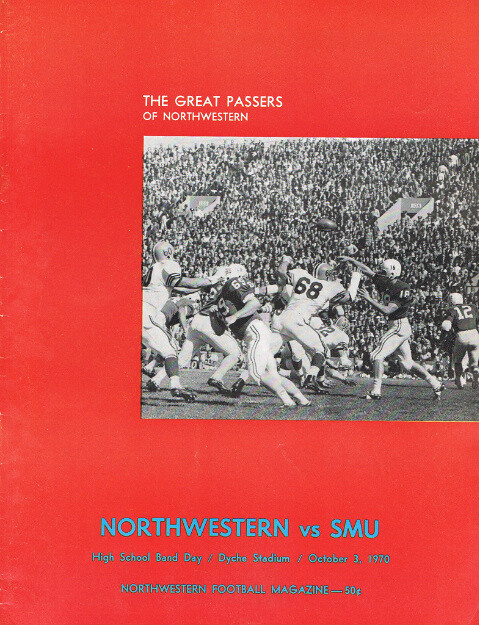This vertical rectangular image is the cover of the "Northwestern Football Magazine" from October 3, 1970, priced at 50 cents. The bright red cover features a black and white action shot in the center, depicting a heated moment in a college football game between Northwestern and SMU. In the photograph, a player, perhaps wearing a number 68 jersey, is seen attempting to intercept a pass while others rush towards the action. The top of the cover is adorned with the title "The Great Passers of Northwestern" in white letters, while just below, it reads "Northwestern vs. SMU, High School Band Day, Dyke Stadium" in blue letters. The background of the photograph reveals a packed stadium, with rows of seats filled with spectators, capturing the electric atmosphere of the game.